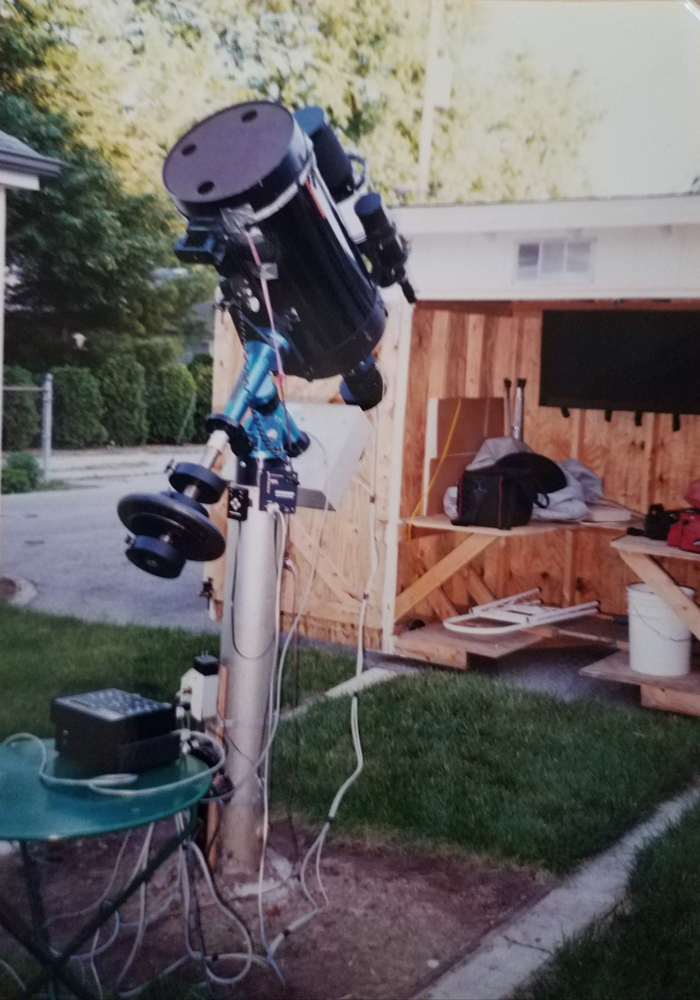This grainy, faded photograph captures an elaborate, large amateur telescope set in someone's grassy backyard. The telescope, made from a giant black canister, is mounted on a sturdy metal pole that's securely set in the ground. It's equipped with various wires connected to a black control box, suggesting it can capture photographs of the sky and adjust lens positioning electronically. Nearby, a plywood shed with open shelves holds a variety of items like a folding chair, a bucket, and other protective covers for the telescope. In the background, there are trees, shrubs, a driveway, and part of a house with a visible roof. The shed, which appears to have a TV mounted on the wall, adds to the well-prepared setup, hinting at the owner's dedication to their astronomical pursuits.